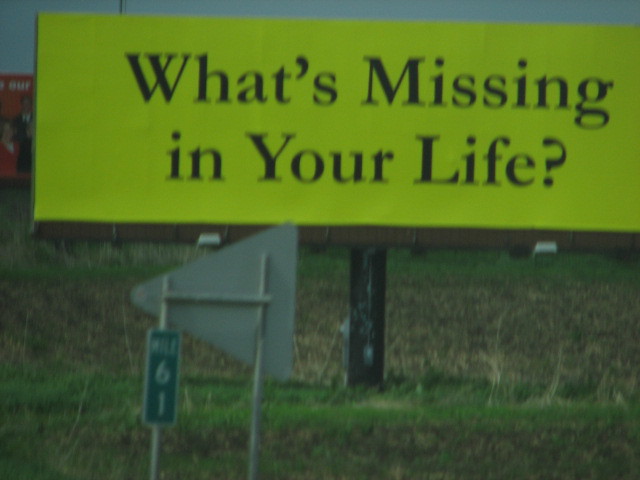The image showcases a large, roadside billboard sign, characterized by its elongated rectangular shape, being approximately three times as wide as it is tall. The back of the billboard is a vivid lime green color, featuring bold black lettering in the center that poses the question, "What's missing in your life?" at its midpoint. The sign is anchored on a solid, thick black pole and is bordered at the bottom by a dark-colored surface, possibly part of the structure's base. Surrounding the billboard is a field interspersed with green and yellow grasses and weeds, along with patches of darker, barren ground. Additionally, the image captures the rear view of a triangular or arrow-shaped road sign, entirely silver, making its front content unreadable. Attached to one of its supporting legs, there is a small, vertical green banner sign that reads, "Mile 61."